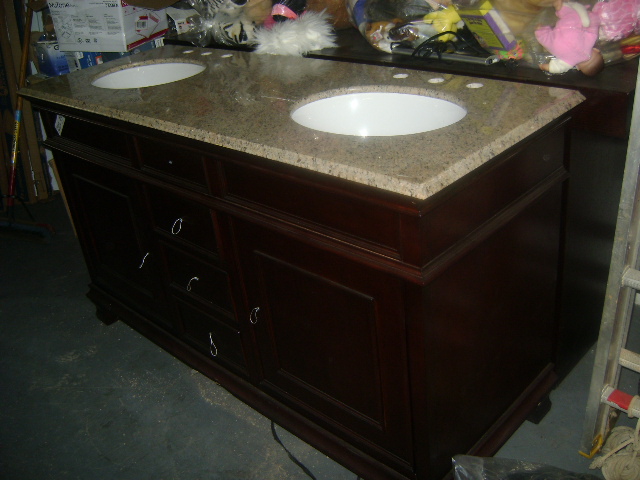This image depicts a dual-sink vanity in a landscape orientation. The sinks are circular and pristine white, standing out against a brownish-gray marble countertop. Behind the sinks, there are three neatly drilled holes in the countertop. The vanity's base and frame are crafted from dark brown cherry wood, providing a rich contrast to the countertop. The cabinetry features five silver handles arranged in a cross-formation across three central vertical doors and two side doors. The vanity is set on an old, green carpet that appears worn and stained with brown spots and dirt. The background reveals a cluttered basement, filled with an assortment of scattered toys, hinting at the space's secondary use for storage and play.